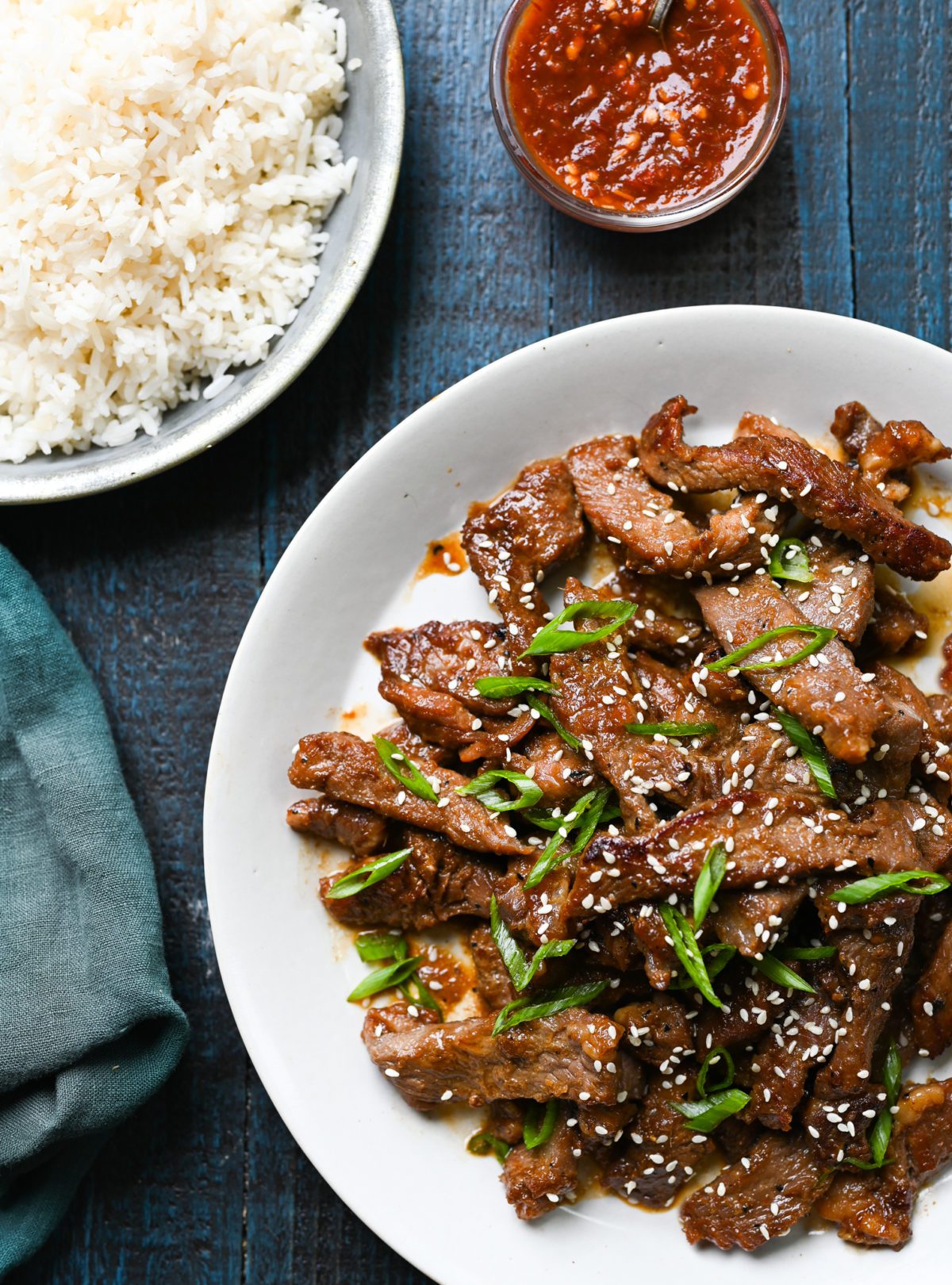In this high-quality image of food on a table, we see two dishes placed on a blue handkerchief. The primary dish, displayed on a white plate with flared edges, consists of tender sautéed beef strips garnished with green onions and sprinkled with sesame seeds. Adjacent to it, on the left side, sits a white bowl containing fluffy white rice. Above these dishes, there is a small cup filled with a vibrant red sauce, possibly a chili or hot sauce, characterized by its larger seeds that resemble those found in chili oil. To the left of the rice bowl, we notice a light blue or green handkerchief. The black table underneath provides a striking contrast that enhances the visual appeal of the food arrangement.